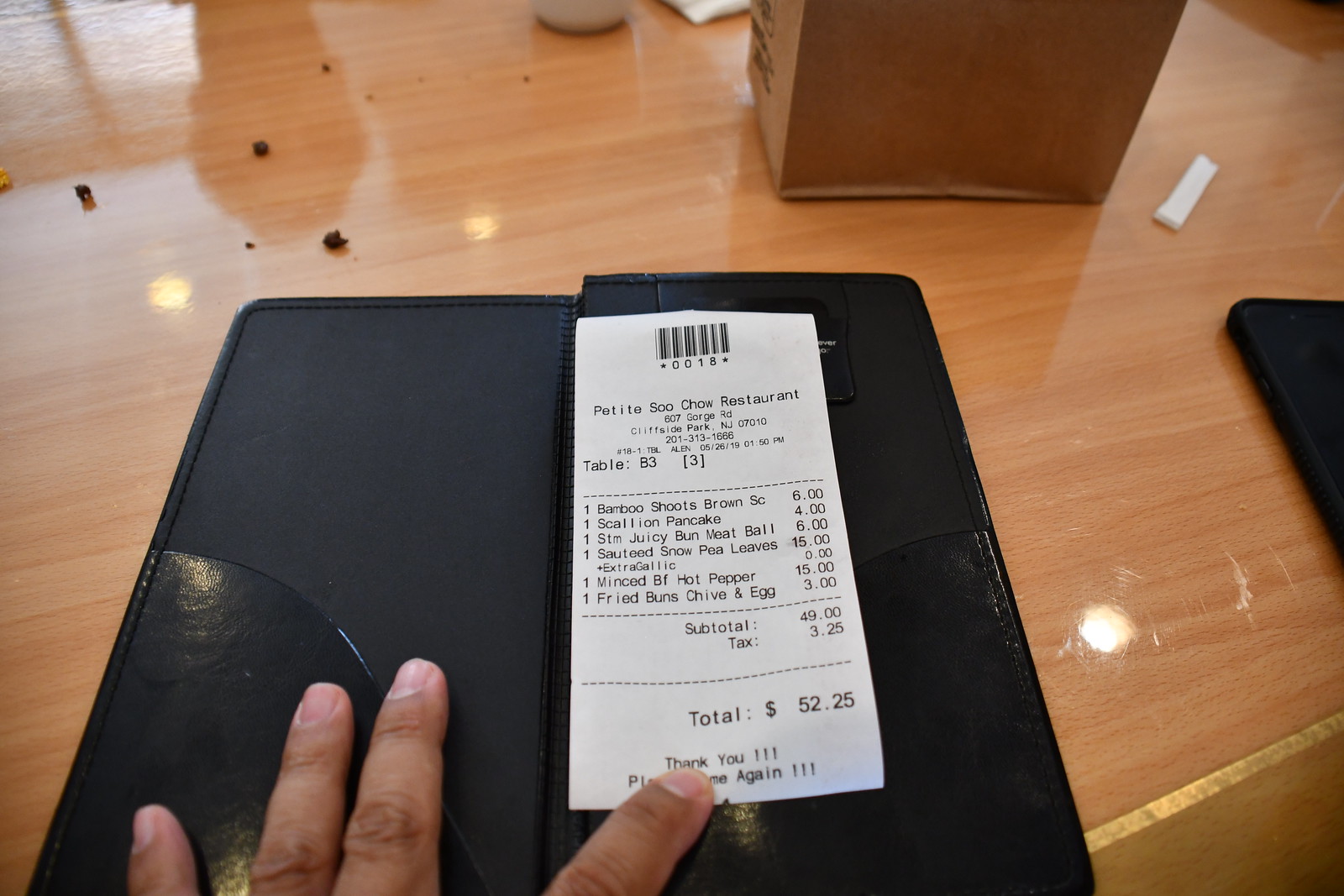A close-up image captures a wooden table. On the table lies an open black wallet, from which a restaurant receipt protrudes. The receipt is from "Petite Sioux Chow," a restaurant located at 607 George Road, Cliffside Park, New Jersey, 07010. A brown-skinned hand is visible in the frame, with only four fingers showing: the pinky, ring, middle, and index fingers. The index finger points directly at the receipt.

The receipt details an order from table B3, itemized as follows:

- **Bamboo Shoot (Brown SC):** $6.00
- **Scallion Pancake:** $4.00
- **Steamed Juicy Bun (Meatball):** $6.00
- **Sautéed Snow Pea Leaves (with extra garlic):** $15.00
- **Minced Beef Hot Pepper:** $15.00
- **Fried Bun (Chive and Egg):** $3.00

The subtotal is listed as $49.00, with a tax of $3.25, bringing the total to $52.25. The bottom of the receipt reads, "Thank you. Please come again."

Surrounding the wallet and receipt, the table shows signs of a recent meal, with small food debris scattered about. A small white piece of paper and a brown bag are also visible on the table, adding context and realism to the dining experience depicted in the image.